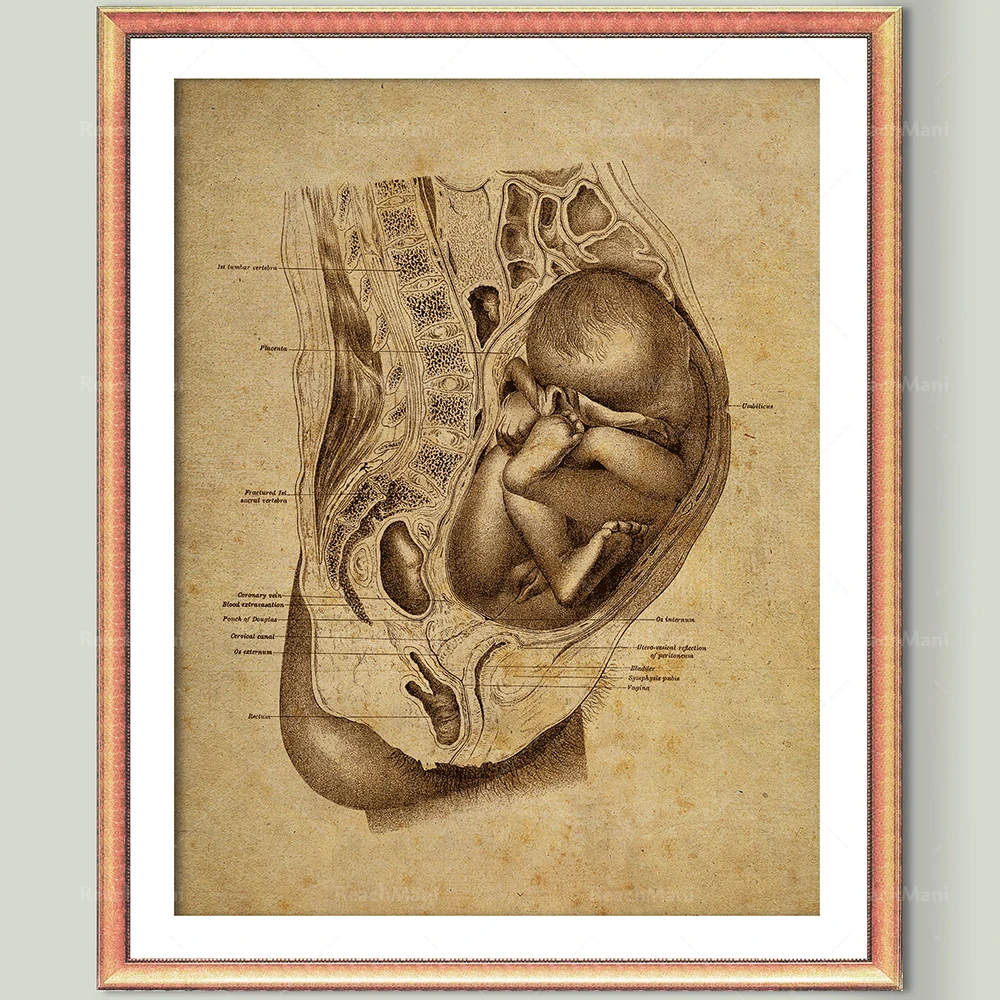The image is a photograph of an old, monochrome scientific diagram displayed on a gray wall. The diagram, which has aged and shows signs of browning, is framed in a brown wooden frame with a white outline. It depicts a detailed cross-section of a pregnant woman's torso, emphasizing the anatomy and the positions of internal organs. The fetus, appearing to be around eight to nine months along in the pregnancy, is shown in a curled-up position within the womb. The diagram includes small, unreadable text that likely labels various organs and anatomical features. There are faint, unreadable watermarks visible on the image, adding to its vintage appeal. Overall, the appearance and detailed representation make it an interesting and informative scientific document.